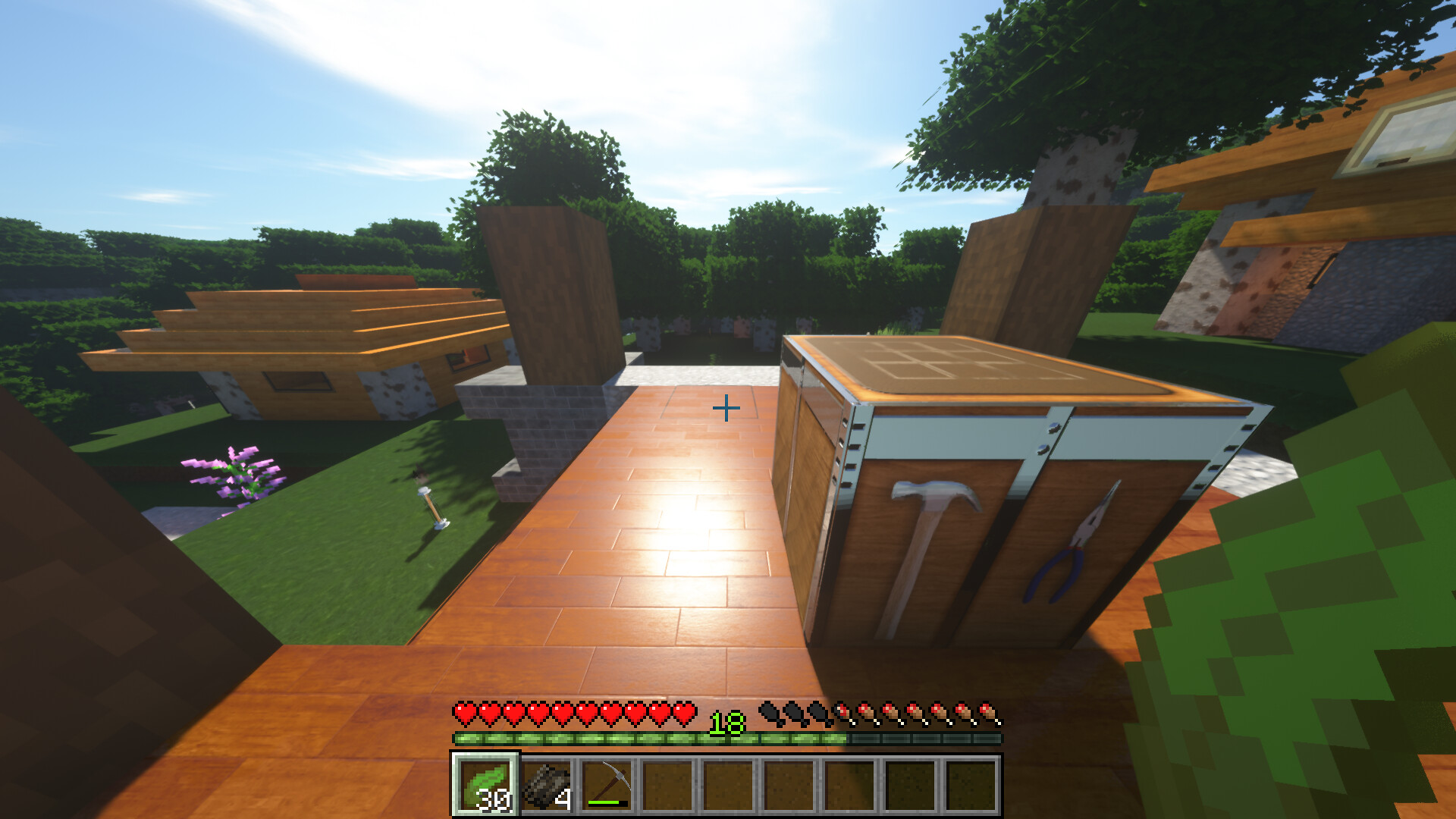This screenshot captures a pixelated scene from a video game, showcasing an environment built with retro-style graphics. The bottom of the image features a red-brick platform, serving as the game's floor, which spans the width of the screen. Dominating the center of the image is a small aiming reticle, resembling a plus sign. Below this, a user interface displays a series of tiny squares, with the first one highlighted, indicating it is selected.

A red-dotted line runs parallel to the row of squares, presumably representing some form of game metric or status. On the left side of the interface, icons representing hearts are displayed alongside the number 18, indicating the player's health or lives. On the right side, there is another set of icons with three missing pieces, though their exact function is unclear.

In the background, towering columns punctuate the end of the platform, flanked by trees, providing a sense of depth. To the left of the scene stands a yellow building with a multi-tiered, stair-step roof. Adjacent to this structure is a plant adorned with purple leaves, adding a splash of color to the otherwise subdued landscape.